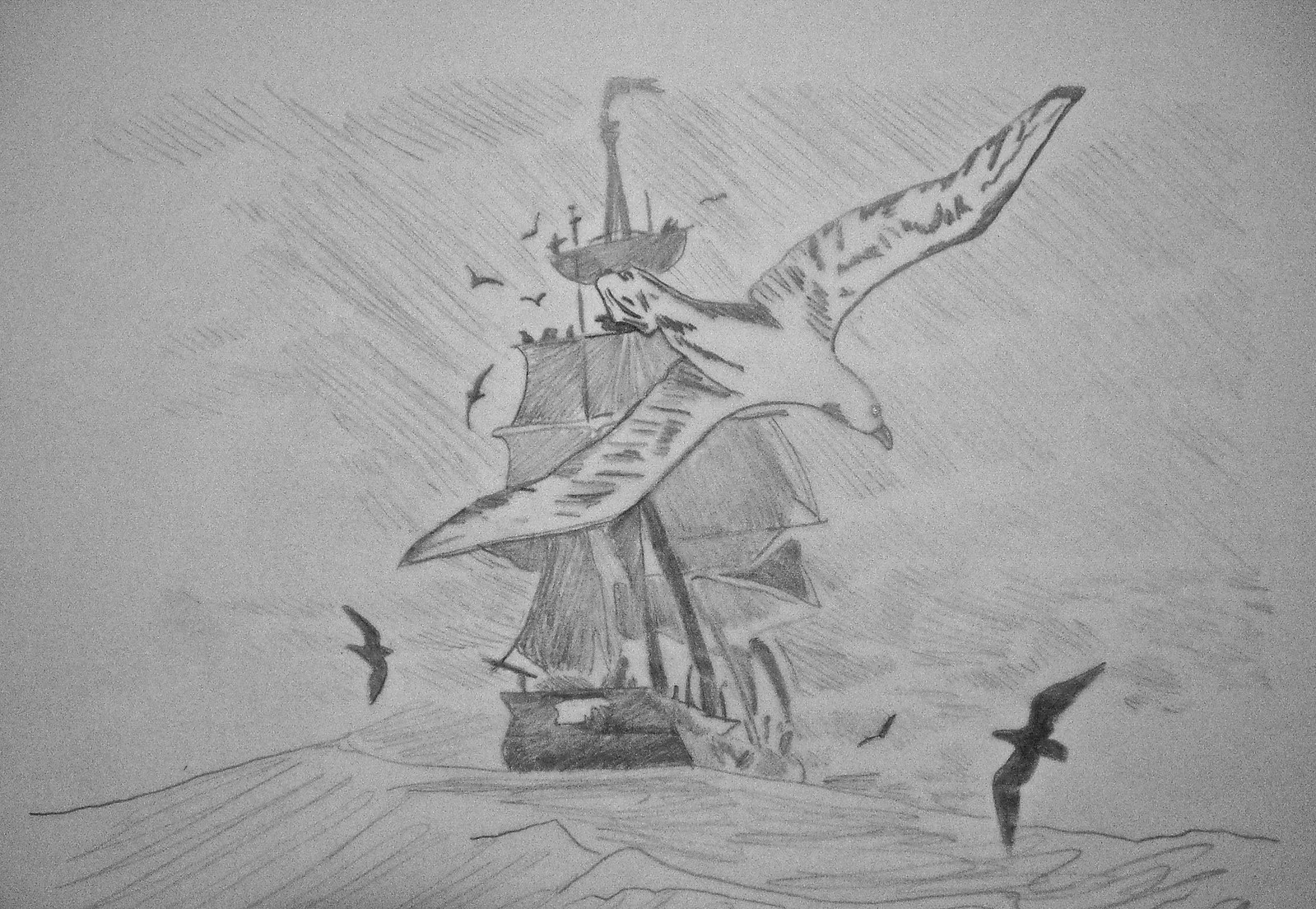A meticulously detailed pencil drawing depicts an old-fashioned sailing ship braving a stormy sea. The ship, with its fully filled sails, cuts through tumultuous waves, conveying movement and intensity. In the foreground, a seagull dives toward the water, its wings outstretched and its beak aimed precisely at the tumultuous sea below. The artist has intricately detailed this seagull, showcasing the texture of its feathers, the sharpness of its beak, and the intensity in its eye. Surrounding the ship, several other seagulls whirl in the stormy sky, rendered as stark black silhouettes that enhance the dramatic scene. This composition skillfully captures the chaos and beauty of nature intertwined with human endeavor.